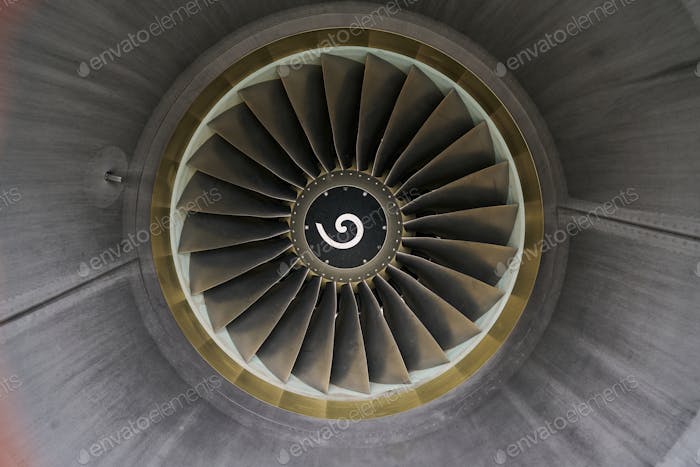The image depicts an industrial-looking, circular ceiling fan with a stationary yet clearly functional blade system. The central area features a distinctive white spiral or swoosh design set against a light brown or tan background, encased within a circular frame of fan blades. These blades extend outward and are set in a white casing, bordered by a gray or brushed steel-like material. Surrounding the unit is a fabric-like texture, possibly sewn, that integrates with the overall design. The entire image is overlaid with a repeating watermark from Envato Elements, text spanning across the image diagonally in a grayish pattern.